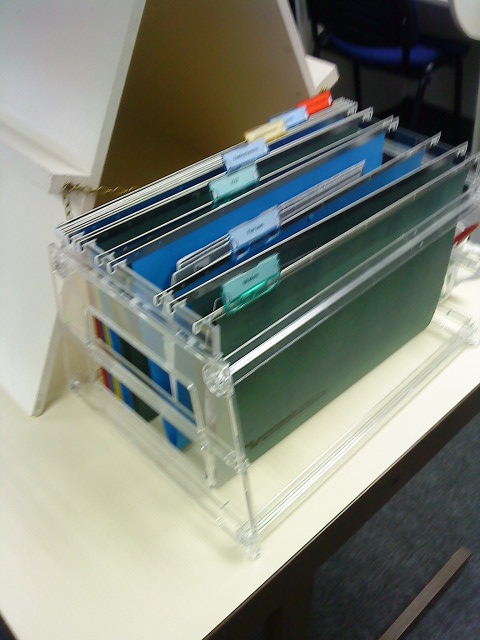This is a slightly blurry home photograph showcasing a clear plastic file organizer prominently positioned on a white desk. The organizer contains an array of colored files, notably green, blue, and black, with tabs in colors including green, blue, yellow, and red. These tabs are efficiently arranged to facilitate easy file identification. Behind the file organizer, there is an A-frame sandwich board sign connected by a chain, although no sign is attached to it. The desk itself is situated in a room where the floor appears to be dark, possibly black or blue. In the background, a white wooden shelf is partially visible, and there might also be a person with blue pants sitting in a dark chair. The overall scene hints at an organized workspace amidst a slightly chaotic environment.